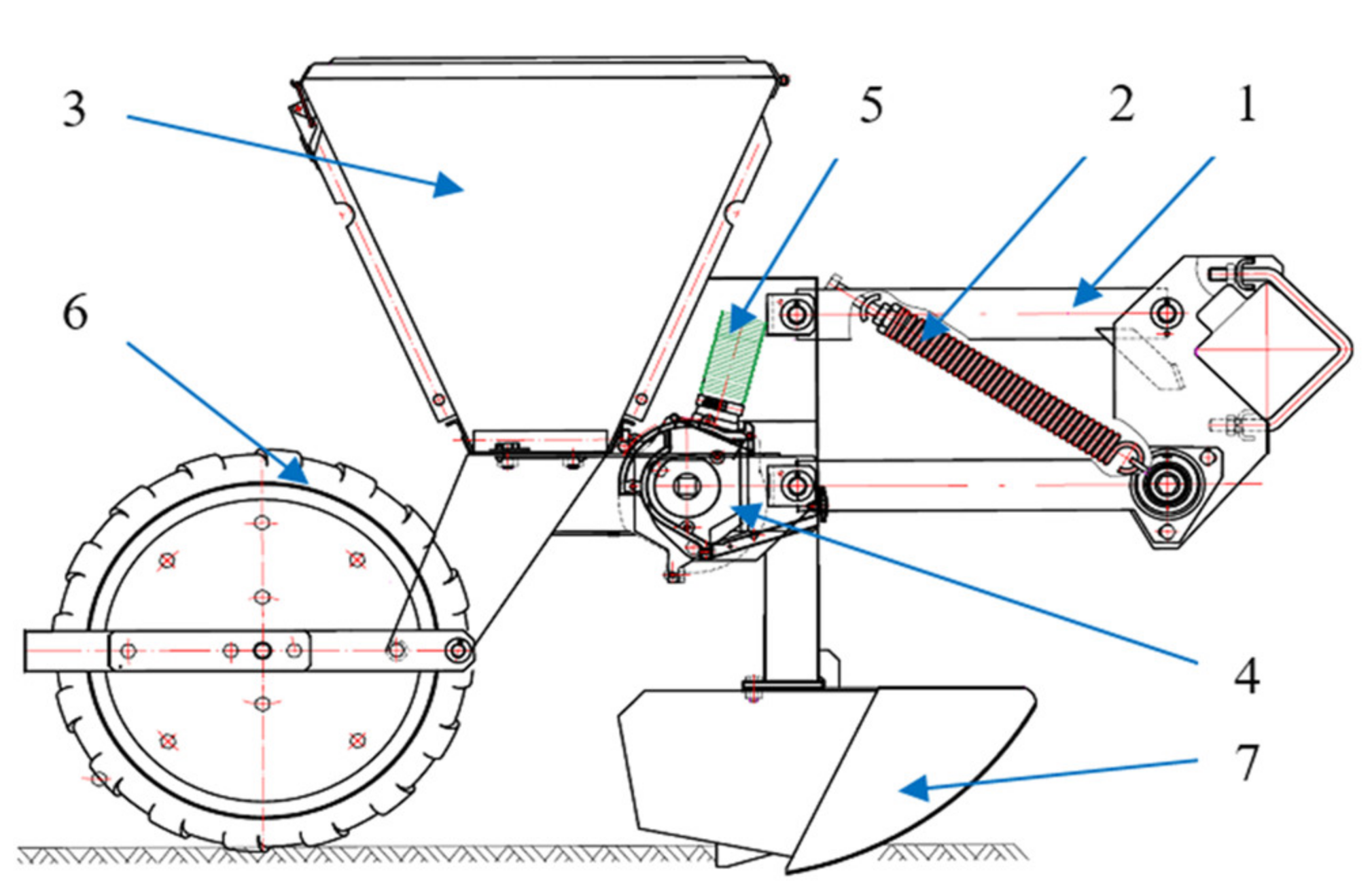The image is a simple yet detailed black and white technical drawing with color accents, depicting a farm seeder machine labeled with numbers 1 through 7. Number 1, identified by a blue arrow, is an arm mechanism likely responsible for moving part 7. Number 2, also highlighted by a blue arrow, points to a large vertical spring at a slant, suggesting it is an essential part of the mechanism. Number 3, indicated by a blue arrow, refers to a large, upside-down triangular hopper where seeds are stored before being sowed. Number 4, pointed out by another blue arrow, resembles a motor essential for the machine’s operation, and sits below number 5, a green rectangle that appears to represent some form of liquid system, potentially for oiling or wetting seeds. Number 6 identifies a large wheel, crucial for both movement and seed compression into the soil. Finally, number 7 appears to be a complex geometric structure incorporating a square and a triangle, likely essential for the seed dispersal mechanism. The diagram, resembling pages out of an operator's manual, includes colored elements and arrows—blue arrows and components in red, green, and orange—on a white background, illustrating the intricate inner workings and layout of the seeder machine.